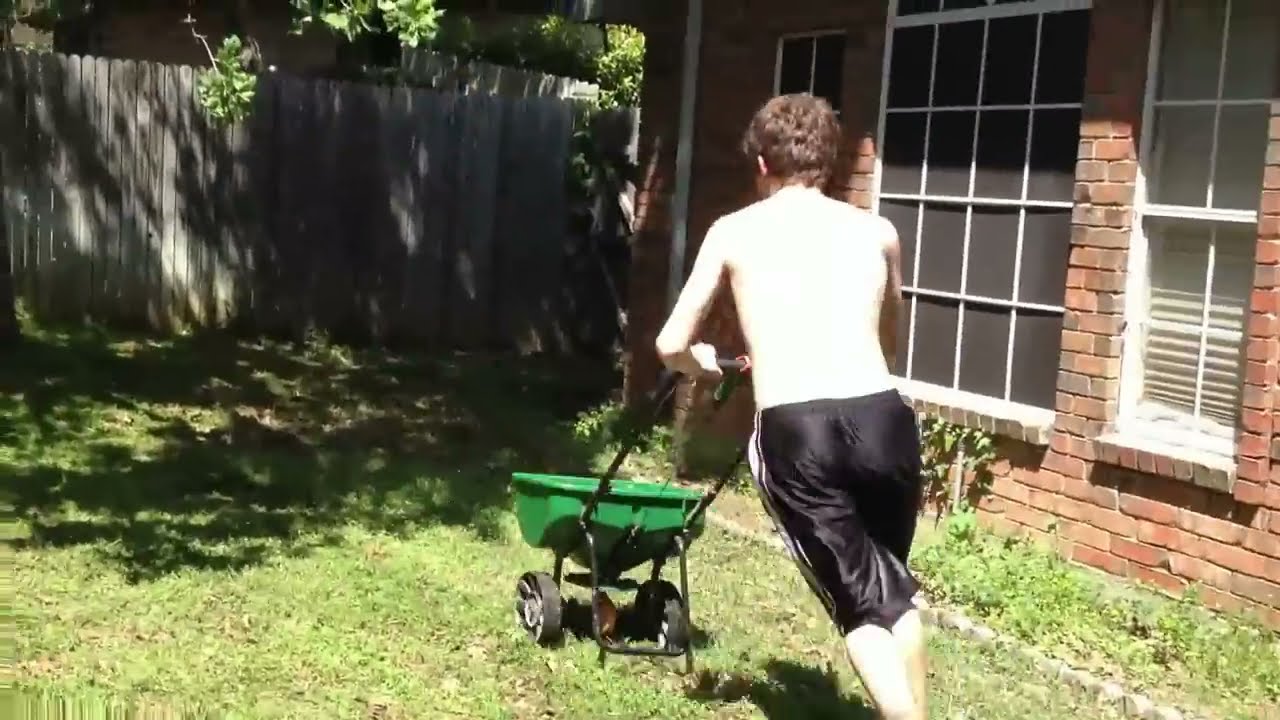A young, shirtless, Caucasian male with short brown hair is pushing a green fertilizer spreader over lush green grass, speckled with patches of brown. He is wearing black basketball shorts and is positioned with his back to the camera, exerting effort as he pushes the spreader, suggesting an action shot. The scene is set in a fenced backyard, where the sun casts shadow and partial sunlight over the grass. To the right is a red brick house featuring white paned windows; one window has visible blinds while the other has a black screen. A drainpipe runs down the end of the house. A flower bed filled with greenery is located in the bottom right corner. In the top left quadrant, a wooden fence is cast in the shadow of a tree, contributing to the shaded area of the yard.